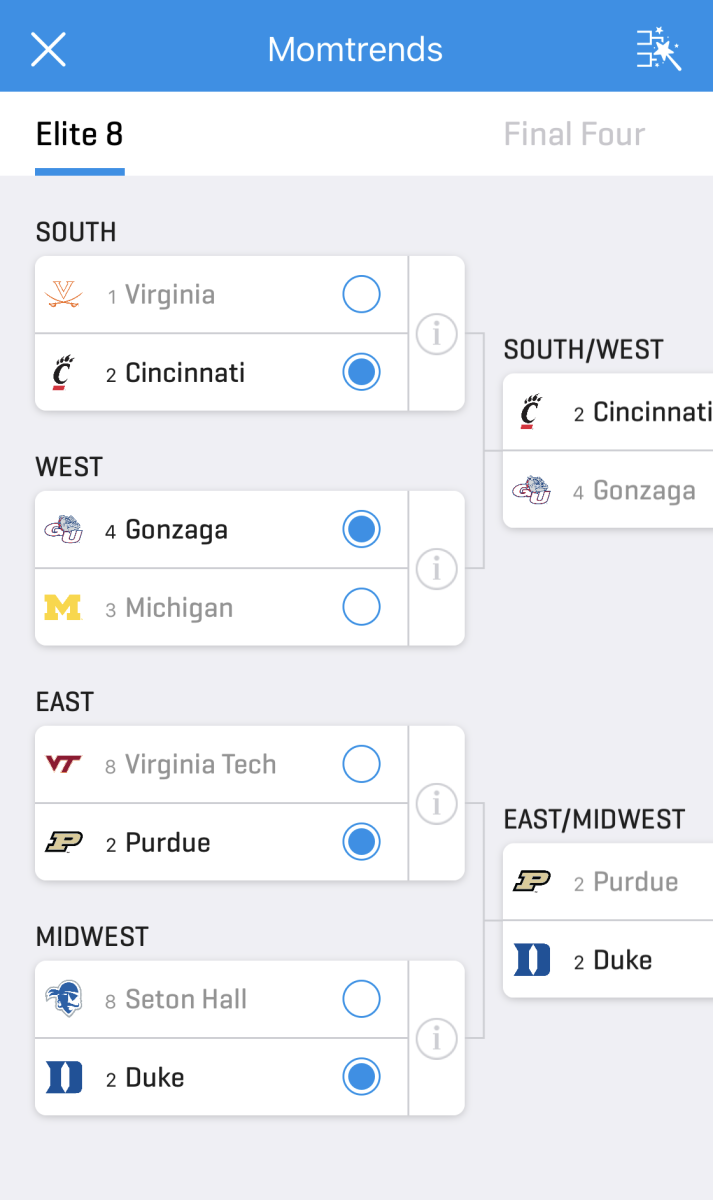The image features a light blue background with the "Mom Trends" logo prominently displayed. On the left, there is an "X" symbol, and to the right, there is a star on a stick resembling a magical wand. At the top, the phrase "Elite Eight" is underlined in blue text. 

The South region includes two labeled circles: Virginia (1) and Cincinnati (2), with Cincinnati's circle shaded blue. The West region shows Gonzaga (4) and Michigan (3), with Gonzaga's circle shaded blue. 

For the East region, Virginia Tech (8) and Purdue (2) are listed, with Purdue's circle shaded blue. In the Midwest region, Seton Hall (8) and Duke (2) are listed, with Duke's circle shaded blue.

There are lines connecting the South and West regions to a section labeled "Southwest," featuring Cincinnati (2) and Gonzaga (4). Similarly, lines from the East and Midwest regions lead to a section labeled "East/Midwest," which highlights Purdue (2) and Duke (2).